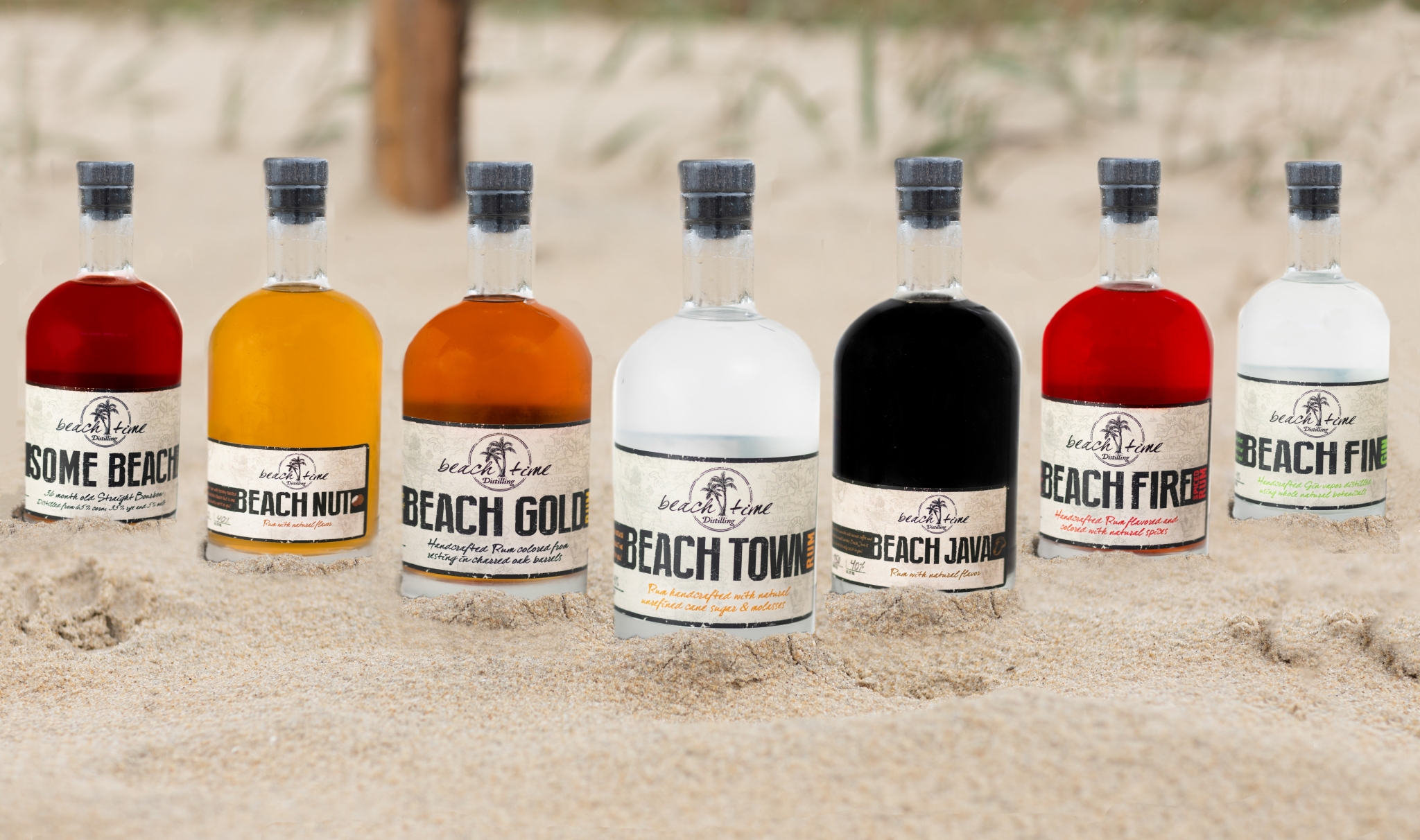A close-up photograph captures seven large bottles of alcohol half-buried in beach sand, lined up side by side with equal spacing under natural light. From left to right, the bottles contain liquids of various colors: the first with a reddish liquid labeled "Some Beach," followed by an orange-colored "Beach Nut," a cherry-colored "Beach Gold," and a clear-colored "Beach Town." Next in line is a bottle with black liquid labeled "Beach Java," another cherry-colored "Beach Fire," and finally, a clear liquid bottle labeled "Beach Fin." The bottles are transparent, topped with black caps, and adorned with labels showcasing names like "Beach Gold," "Beach Town," "Beach Java," and "Beach Fire." The background features blurry grass and a wooden pole, emphasizing the beach setting.